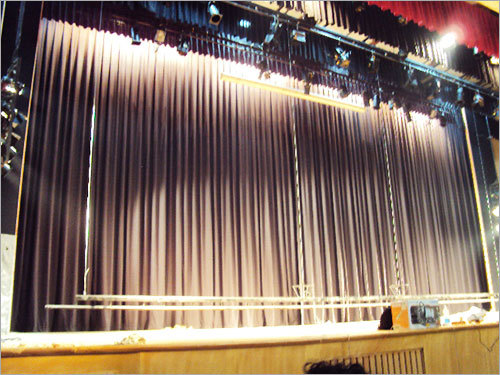The image depicts a stage, possibly located in a school or theater, framed by prominent yellow curtains that extend fully from the top to the bottom of the stage. Above these curtains, a smaller maroon curtain is visible, positioned in the top right corner. The stage is well-lit by numerous vertically oriented stage lights, some arranged along both the top and sides of the stage, enclosed in black lampshades. The stage floor appears to be wooden and slightly elevated. On the right side of the stage, there are some props or equipment, including a yellow bag and a gray rectangular object. The scene features a bit of someone's hair at the bottom center-right, suggesting an onlooker is present. Overall, the setting and lighting create a well-defined stage environment, prepared for performances or events.